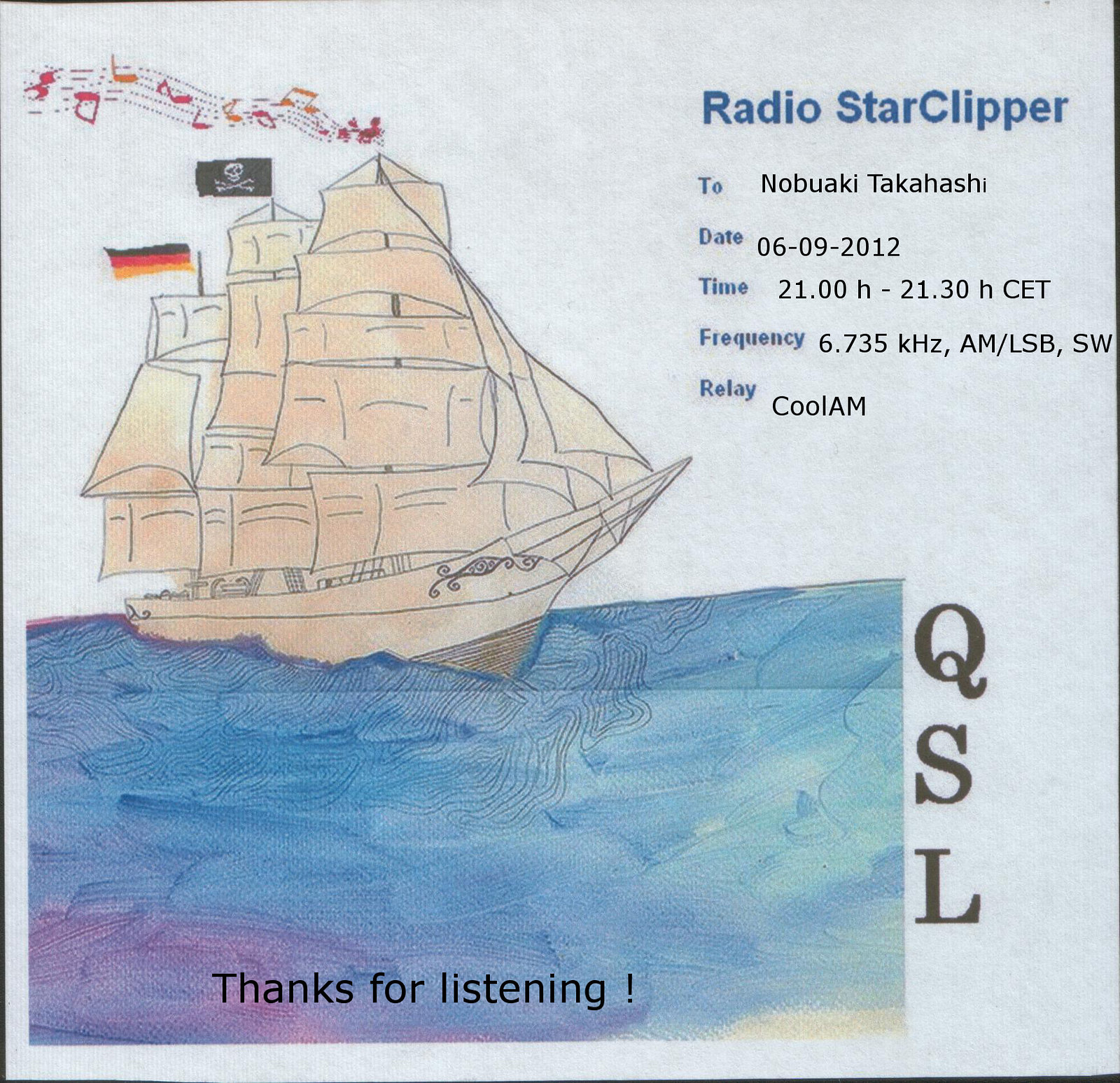The image is a detailed watercolor painting of an old-timey pirate ship sailing on a light blue and white ocean, with hues of purple. The ship is depicted with three masts adorned with a variety of flags, including a pirate flag at the top and a German flag with horizontal black, red, and yellow stripes. Musical notes appear to float off the top of the front mast, adding a whimsical touch. The entire artwork is printed on textured, napkin-like paper with a slightly black background visible in some areas. 

The key details from the page are organized around the painting: at the top right in blue text is "Radio Star Clipper," and below it reads "To Nobuaki Takahashi." Further down, specific information is listed: the date 06-09-2012, the time 21:00 – 21:30 HCET, the frequency 6.735 kHz AM/ LSB SW, with the relay station noted as "Cool AM." Towards the bottom, black text states "Thanks for listening," and the phrase "cute as hell" appears to the right of this. The bottom right corner features the text "QSL," aligning vertically from top to bottom.